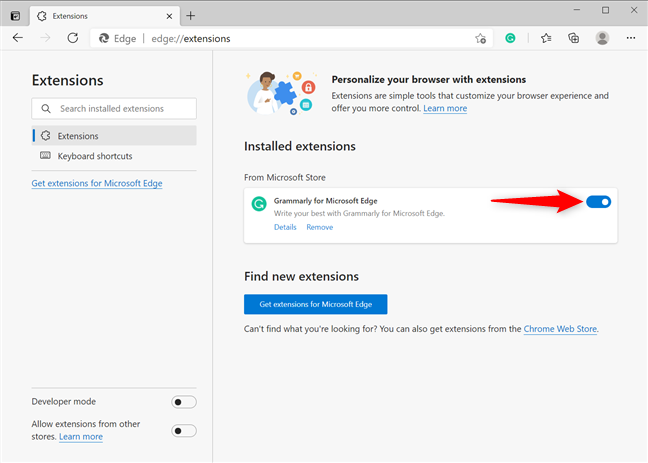The screenshot features the Microsoft Edge browser's Extensions page set against a gray background. At the top of this page, notable elements include navigation icons like a left arrow, right arrow (which appears more gray than black), and a refresh symbol. The address bar displays "edge://extensions" while showcasing a box to search installed extensions, marked by a magnifying glass icon.

The central area of the page consists of a gray box containing multiple sections. Firstly, it highlights the Extensions workspace with a puzzle piece icon and options like "Keyboard shortcuts" and "Get extensions from Microsoft Edge" in blue text.

Below, there are toggle switches for "Developer mode" (set to off) and "Allow extensions from other stores" with a "Learn more" link in blue, again set to off.

A section titled "Personalize your browser with extensions" describes how extensions can customize the browser experience and provides further control, with another "Learn more" link in blue.

Moving to the installed extensions part, it shows "Grammarly for Microsoft Edge," indicating that the extension is currently active. Associated actions include "Details" and "Remove," both in blue text, accompanied by a red arrow pointing to a toggle switch turned on.

At the bottom, under "Find new extensions," there's a prominent blue button labeled "Get extensions from Microsoft Edge." An additional message reads, "Can't find what you're looking for? You can also get extensions from the Chrome Web Store," with "Chrome Web Store" highlighted in blue.

This descriptive detail captures the essence and functionality visible within this Microsoft Edge Extensions page screenshot.